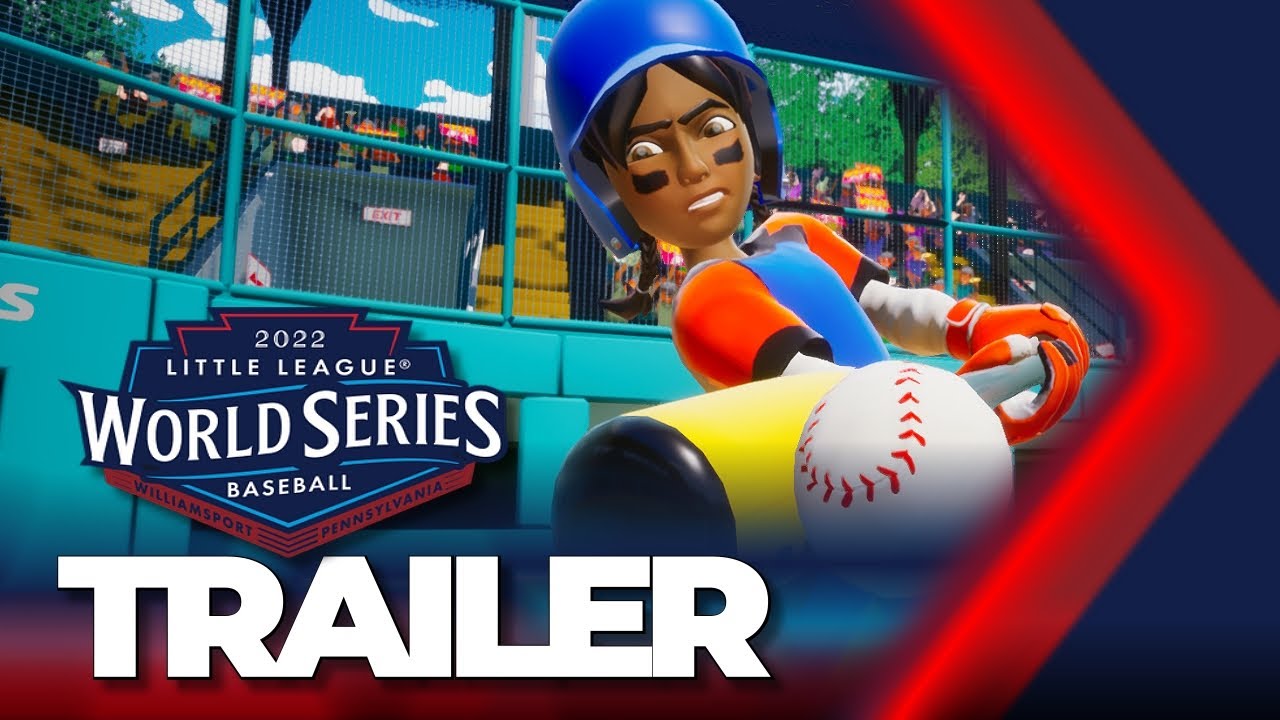The image is an advertisement for the "2022 Little League World Series Baseball," set in Williamsport, Pennsylvania. It appears to be a trailer for a video game, highlighted by the large, bold white letters spelling "TRAILER" at the bottom left. Just above this word, there's a logo featuring the text "2022 Little League World Series Baseball Williamsport, Pennsylvania" in a chevron-shaped design.

Dominating the scene, a cartoonish black female character is in mid-swing with a yellow baseball bat, poised to hit an incoming baseball. She is equipped with a blue helmet and a blue jersey with red or orange sleeves, layered over a white long-sleeve shirt and matching orange or red gloves. The background showcases a packed stadium filled with spectators, creating a vibrant, tense atmosphere. An eye-catching red arrow extends from the top right side of the image, swooping downward and exiting off the frame, emphasizing the motion and direction of the swing. The entire scene underscores the energetic and competitive essence of the game, reinforcing the impression of an engaging sports video game.